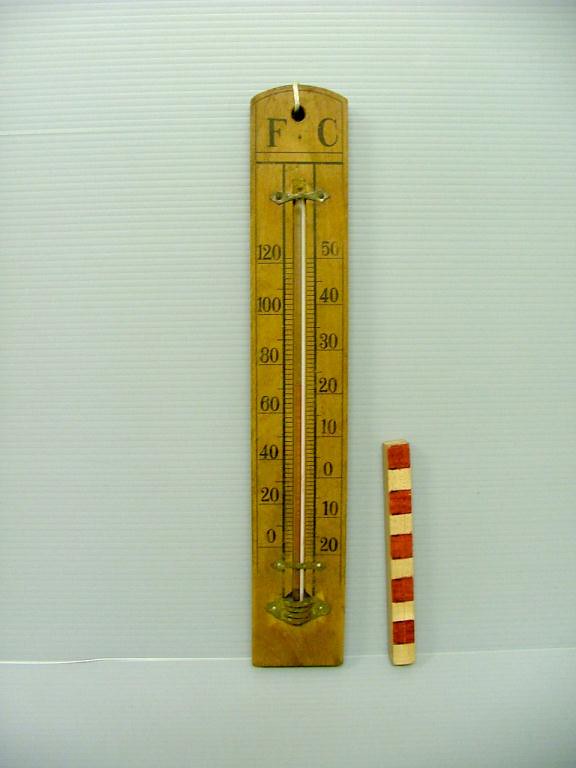A detailed view of an antique wooden thermometer, characterized by its elongated rectangular shape with a rounded edge at the top. A black hole at the apex houses a piece of white string threaded through it. Below, the left side is labeled with a capital "F" (Fahrenheit), progressing in decrements from 120 to 0 degrees. The right side, marked with a capital "C" (Celsius), ranges from 50 to -20 degrees. The thermometer's white central line is fastened to the wooden base by aged, brass-colored braces, with rusted bolts securing it at the top. Additional braces at the bottom are similarly brass-colored but feature shiny yellow bolts. To the right of the thermometer, a small wooden post adorned with red and yellow squares stands, matching the height of 10 degrees Celsius on the scale. The background is a light green wall with horizontal lines that resemble the pattern of a window. Both the thermometer and the post rest on a solid surface that is the same hue as the wall.